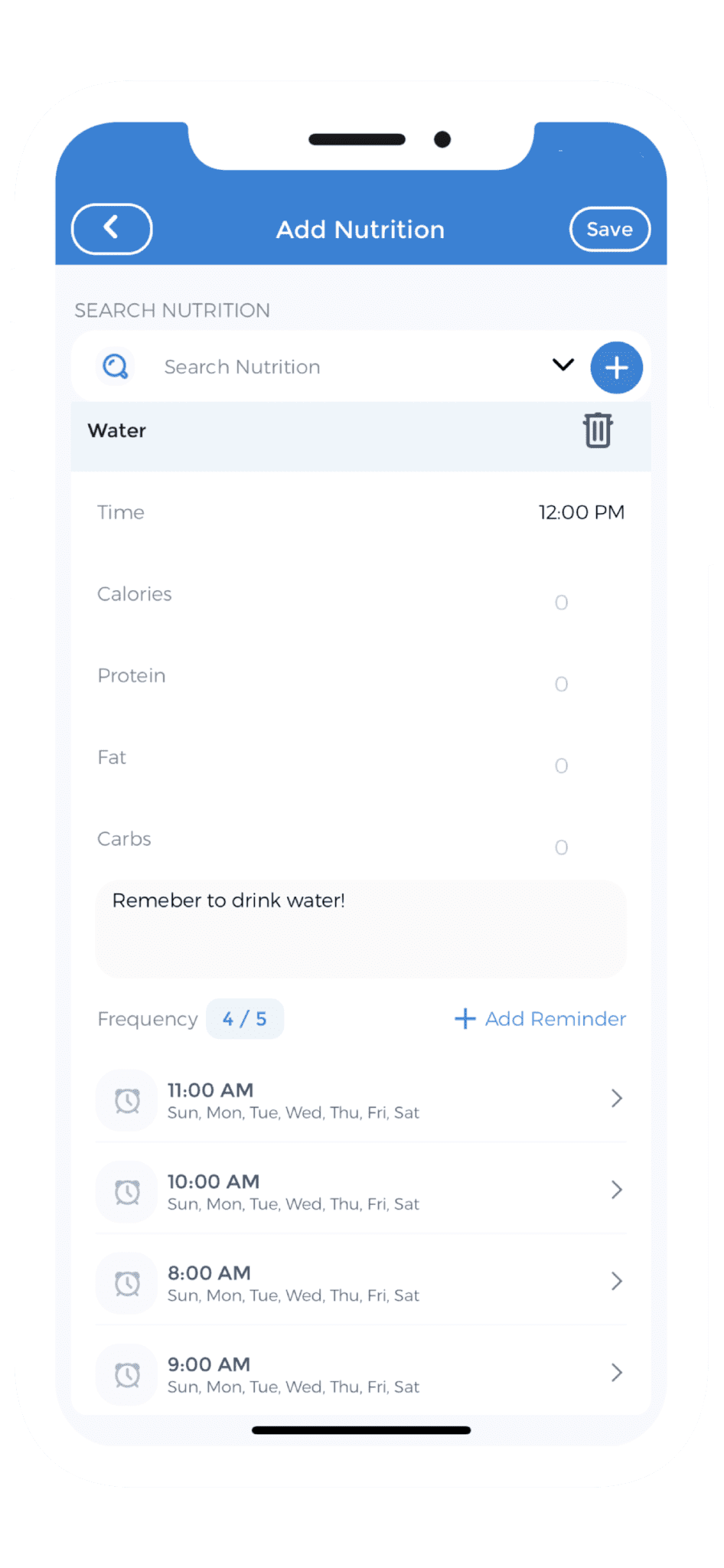The screenshot depicts a mobile app interface, likely from an iPhone, with a clean and user-friendly design predominantly featuring a light blue background. At the top center of the screen, a heading reads "Add Nutrition" in white font. On the top left corner, there is a back button, while on the top right corner, a blue pill-shaped button labeled "Save" is present.

Beneath the heading "Add Nutrition," there is a search input field marked "Search Nutrition," accompanied by a magnifying glass icon and a downward-pointing drop-down arrow to its right. Adjacent to this arrow is a circular plus icon. Below the search field, the word "Water" is listed with a trash can icon to its right, allowing for deletion.

Further down, the interface showcases a section with a white background detailing nutritional information under the headings: "Time" (set to 12 p.m.), "Calories" (at 0), "Protein" (at 0), "Fat" (at 0), and "Carbs" (at 0).

Amid this section, a message box prompts the user with "Remember to Drink Water." Below this prompt, a status displays "Frequency, 4 out of 5," paired with an option labeled "Plus Add Reminder" on its right. Listed underneath are scheduled alarms: 11 a.m., 10 a.m., 8 a.m., and 9 a.m., strategically placed to aid in managing the user's nutrition and hydration throughout the day.